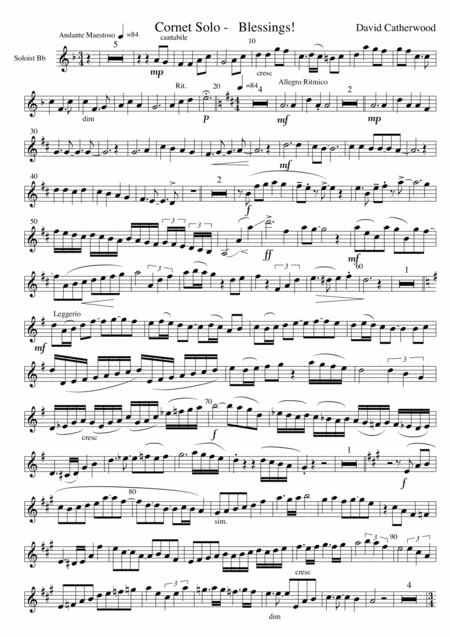This image is a scan of a piece of sheet music titled "Cornet Solo: Blessings" by David Catherwood. The sheet is longer than it is wide and has a white background. At the top of the image, the title "Cornet Solo: Blessings" is clearly printed in black text, with the composer's name, David Catherwood, positioned to the right. Below this heading, there are 13 horizontal lines of music extending from the right to the left side of the page, each beginning with a treble clef. These lines are populated with black music notes, including both filled and open noteheads. Additional musical notation is present below these lines. The notes and symbols are all rendered in black, and the image is devoid of any other text except for the musical notation and the title information at the top. Repetitive musical themes are evident throughout the sheet, contributing to its overall composition.